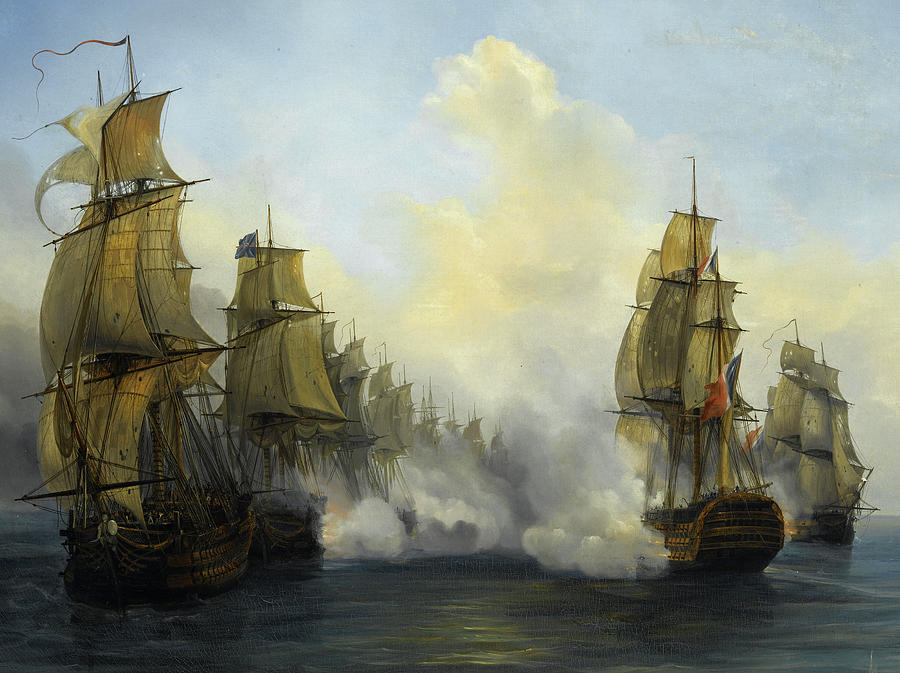This oil painting vividly depicts an intense 1800s sea battle between two lines of old wooden sailing ships with billowing white and off-white sails. The scene is set amidst a cloudy sky and a smoky battlefield, with cannons firing and bursts of smoke filling the air. The ocean appears crisp yet slightly murky, with a greenish-blue tint to the water. The ships, resembling frigates, are equipped with multiple masts and numerous sails. The vessels extend all the way to the horizon, with a hint of national identity shown by a vague flag featuring blue, white, and red colors on one of the ships. Despite the fierce battle evidenced by the heavy smoke and cannon fire, no sailors are visible, emphasizing the grandeur and scale of the ships themselves as they clash for dominance over the turbulent waters.